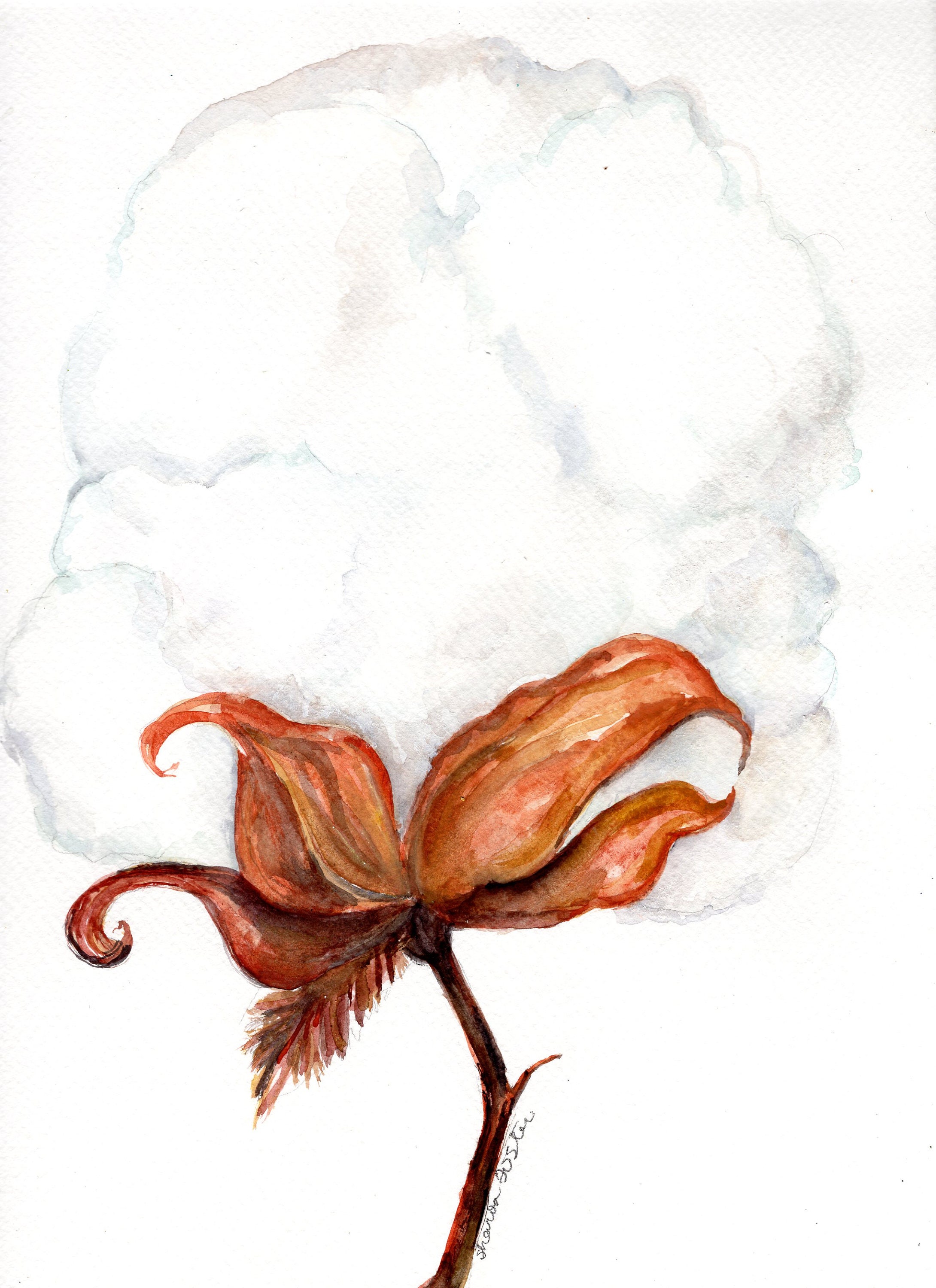This image is a watercolor painting depicting a cotton plant. The background is white, highlighting the detailed foreground. The main focus of the painting is a large, fluffy white cotton ball, reminiscent of a cloud or cotton candy. Subtle shades of blue, green, gray, and white add depth to the cotton, giving it a somewhat ethereal quality. The cotton ball sits atop a rust-colored, brownish stem that stands out sharply against the white backdrop. On the side of the stem, there is cursive writing, possibly the artist's signature, which reads "Sharda Jester" or "Sharon Jester." Accompanying the stem are four petals in varying shades of brown and orange, adding a warm, earthy contrast to the cool tones of the cotton ball. The overall impression is of a delicate plant, captured beautifully through muted, expressive watercolor strokes.